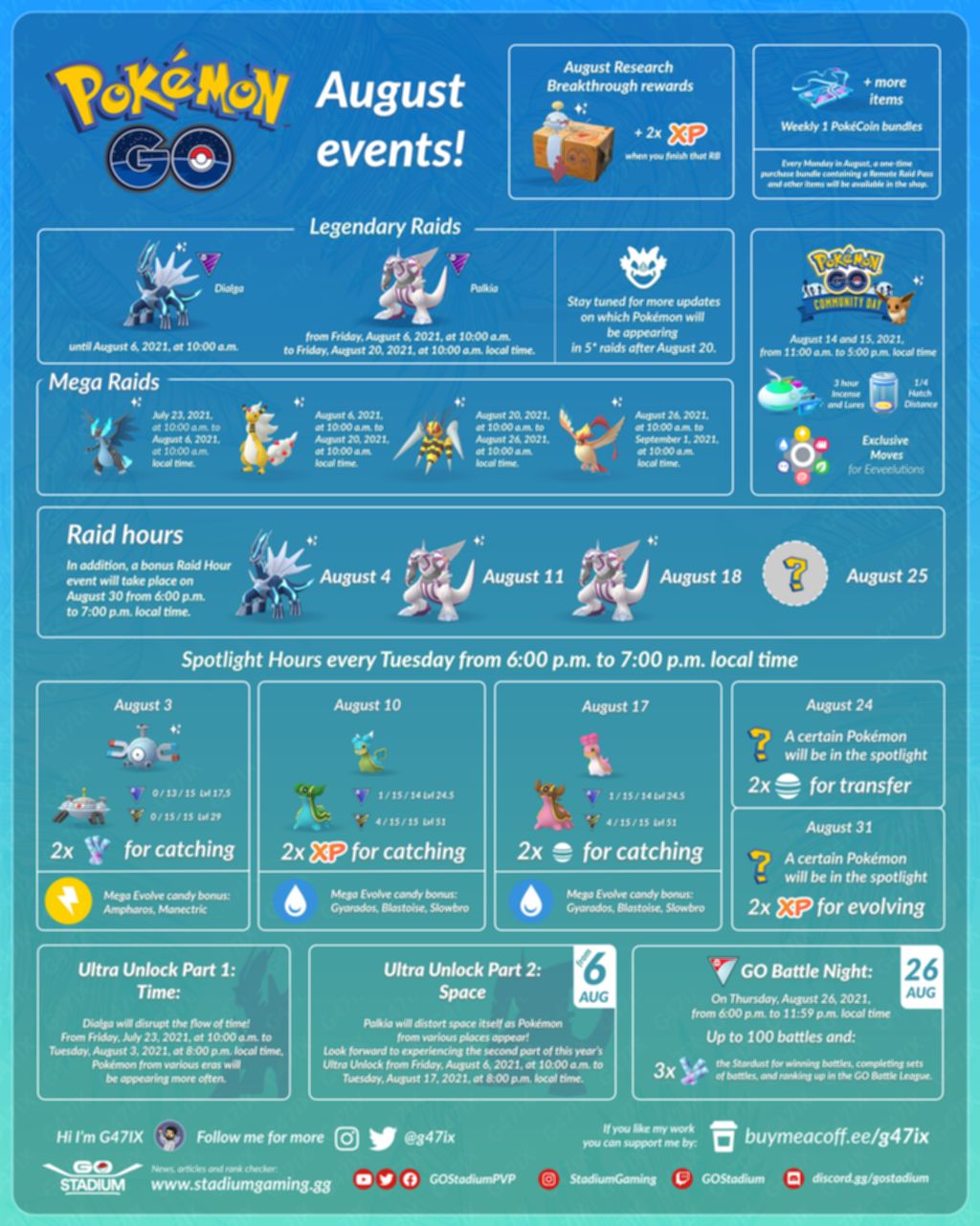**Infographic Description: Pokémon Go August Events**

The infographic presents a comprehensive overview of Pokémon Go events scheduled for August. The background gradient transitions from a serene sky blue at the top to a refreshing sea green at the bottom, creating an inviting and vibrant backdrop.

At the top, the title "Pokémon Go August Events" is prominently displayed, featuring the Pokémon Go logo for brand recognition. Below the title, key features of the month's events are highlighted:

1. **August Research Breakthrough Rewards**: Accompanied by text indicating a 2x XP bonus and an image of a loot box, signaling valuable rewards for players.

2. **Weekly 1-Pokémon Coin Bundles**: Icons illustrate these bundles, indicating additional items that players can obtain on a weekly basis.

3. **Legendary Raids**: This section highlights various legendary Pokémon available for raids, providing options to participate in exclusive events and earn rare characters.

4. **Mega Raids**: Similar to the Legendary Raids, this segment showcases opportunities to win additional powerful Pokémon through mega raids.

5. **Pokémon Go Community Day**: Important community engagement events with options for participation and special bonuses.

6. **Raid Hours**: Specific raid events are outlined, including a special bonus Raid Hour on August 30th from 6 PM to 7 PM local time, along with raid events on August 4th, August 11th, August 18th, and August 25th.

7. **Spotlight Hours**: Spotlight hours occur every Tuesday from 6 PM to 7 PM local time, with distinct activities planned for August 3rd, 10th, 17th, 24th, and 31st.

8. **Special Campaigns**: This section highlights significant events such as Ultra Unlock Part 1, Ultra Unlock Part 2, and Go Battle Night.

The bottom of the infographic provides ways to follow Pokémon Go August events through different social media platforms, encouraging players to stay updated via Instagram, Twitter, Facebook, and more.

This detailed infographic serves as a guide for Pokémon Go enthusiasts to navigate through the exciting events and activities happening throughout August.